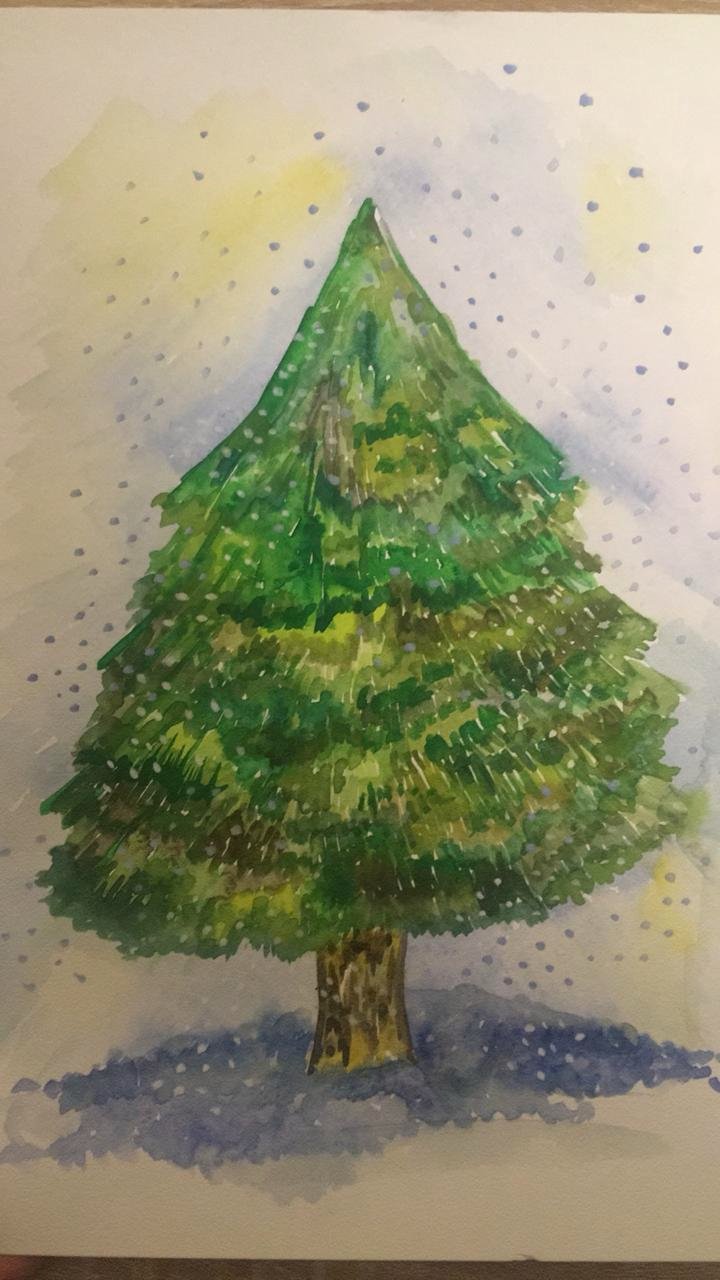A highly detailed and evocative piece of artwork captures a vibrant green tree standing resiliently amidst a winter landscape. The ground surrounding the tree is blanketed in pristine white, clearly symbolizing a thick layer of snow. Despite the wintry setting, the tree—a likely pine based on its green foliage—remains lush and verdant. Delicate white dots scattered throughout the scene artistically represent falling snowflakes, further emphasizing the cold atmosphere. What intrigues the viewer most is the area beneath the tree, tinted in a mesmerizing purple hue, possibly indicating a shadow cast upon the snow. This contrast highlights the tree's dark brown trunk, grounding it firmly in the snowy scene, while the green needle-like leaves offer a striking juxtaposition to the winter elements.